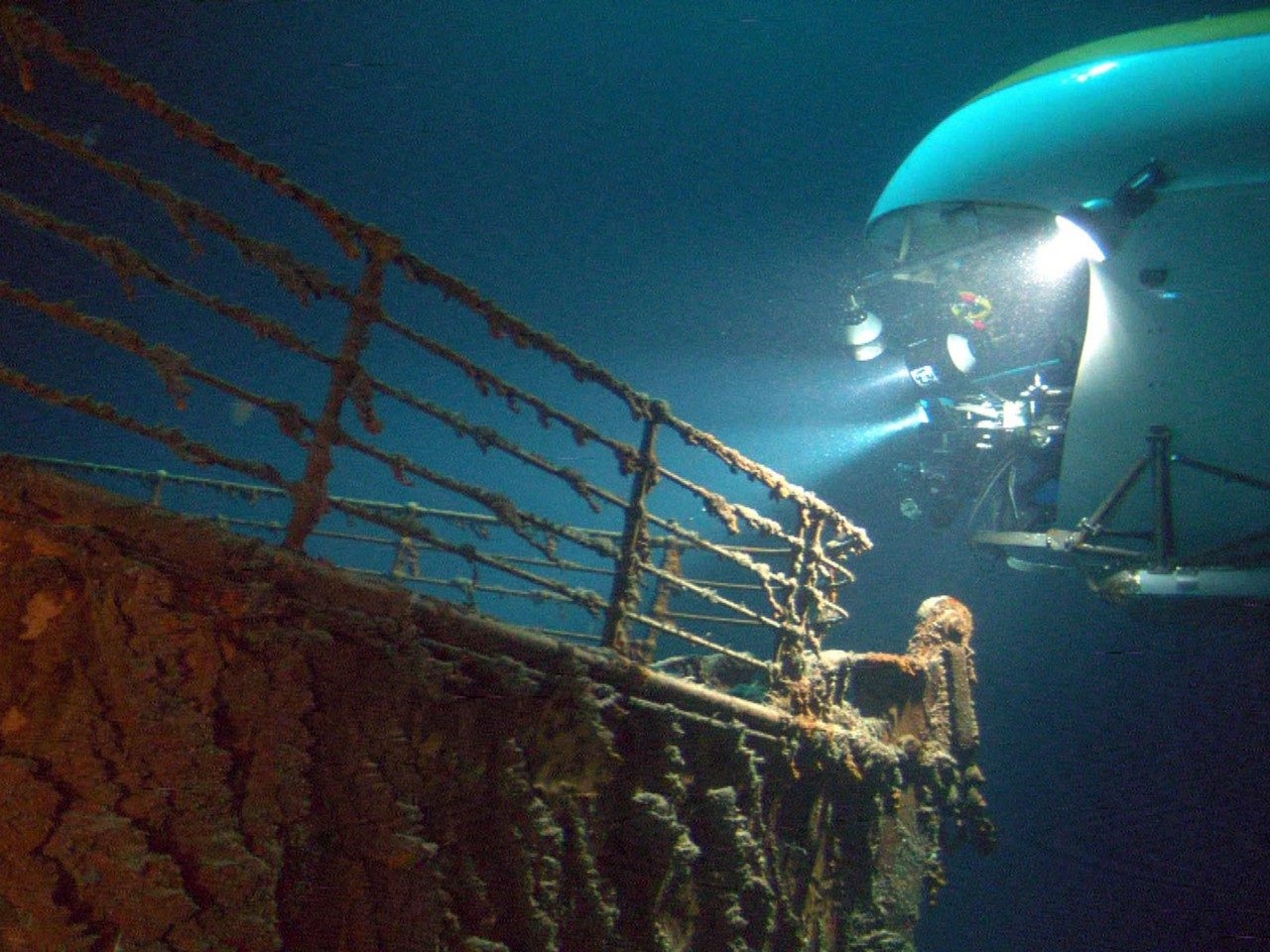The undersea photograph captures a deep-sea submersible illuminating a shipwreck with its powerful lights. Clearly visible through the submersible's windows are crew members and an array of sophisticated equipment. The focal point of the image is the shipwreck, heavily encrusted with rust and algae, which strongly suggests it might be the ill-fated RMS Titanic. Prominently featured is what appears to be the tip of the bow, complete with a deteriorated deck railing that curves back in a familiar trajectory reminiscent of the iconic scene from the Titanic movie where a couple famously poses at the ship's prow. The hauntingly beautiful wreckage is bathed in the submersible’s lights, highlighting the extensive corrosion and marine growth that now blankets this once-majestic ocean liner.